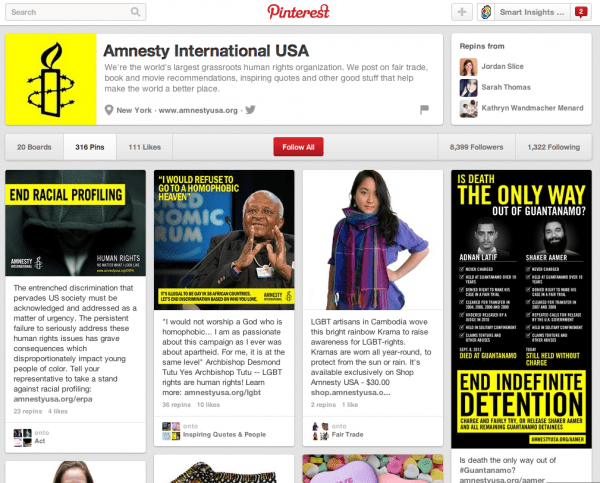The image depicts the homepage of the Amnesty International USA website, which proudly identifies itself as the world's largest grassroots human rights organization. The website, based in New York and accessible at www.amnestyusa.org, features a variety of content aimed at fostering a better world. One can find recommendations for Fairtrade books and movies, inspiring quotes, and various other uplifting and informative postings.

On the right side of the page, there are repins accompanied by the names and pictures of different individuals. Below these, a series of impactful stories are prominently displayed. The first story, titled "End Racial Profiling," features a striking yellow heading set against a black background. Following it is a compelling narrative headlined as "I Would Refuse to Go to a Homophobic Heaven." Another key story highlights LGBT artisans in Cambodia. Finally, there's a powerful piece questioning, "Is Death the Only Way Out of Guana, Montana?" which addresses the urgent need to end indefinite detention. A small Twitter link is also present, suggesting engagement on social media.